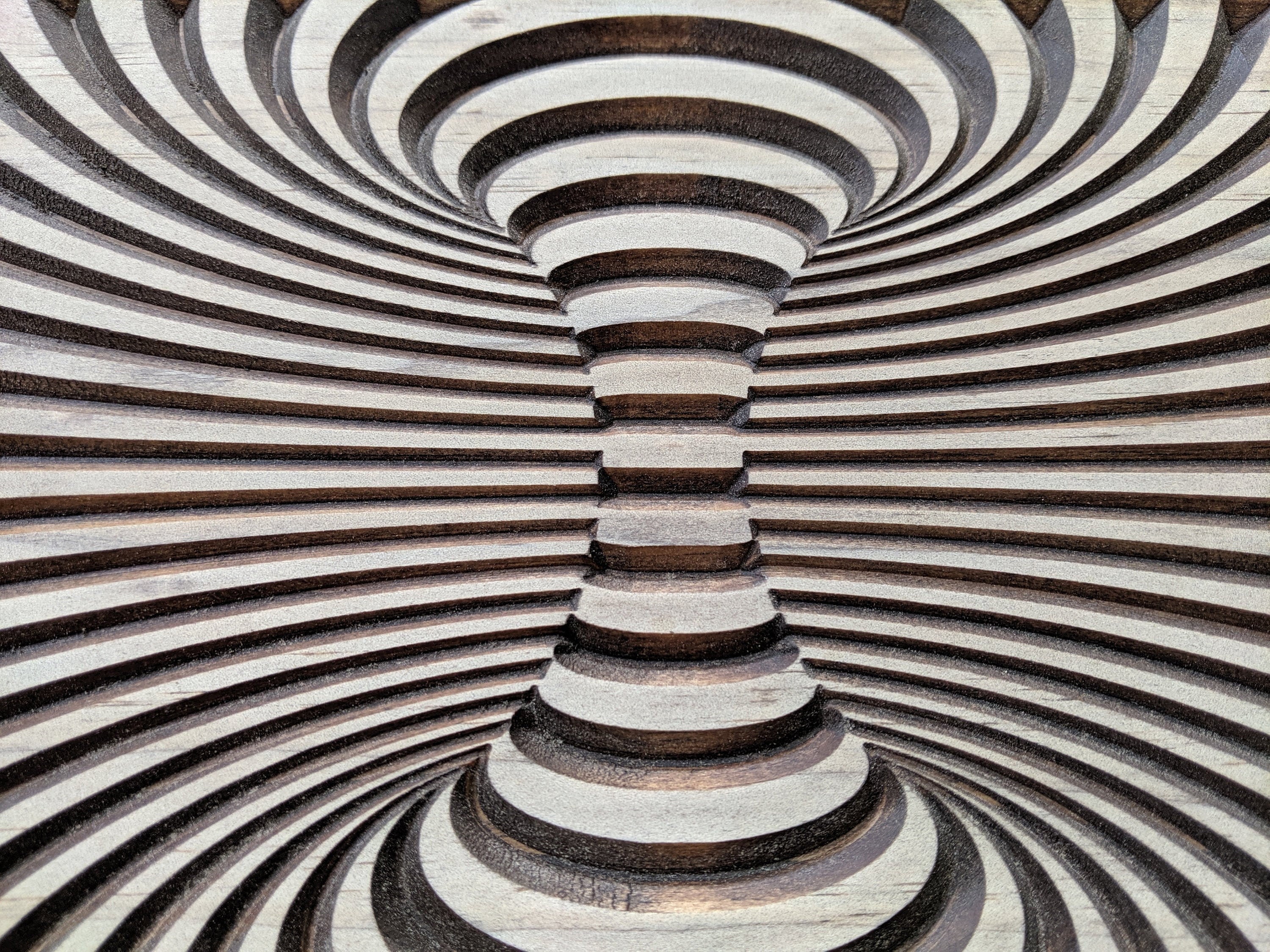This intricate black, white, and gray image gives the illusion of a room in perpetual motion. At its core is a central column that resembles a reverse hourglass or a tornado, expanding outward at both the top and bottom while narrowing dramatically in the middle. Surrounding this column are multiple concentric rings or horizontal stripes, each maintaining consistent thickness. These rings appear to be either painted, drawn, or carved, and wrap around the entire scene, amplifying the sense of rotation. The rings and the column interact in such a way that they seem like extensions of each other, creating an optical illusion of swirling or spinning motion. The use of varying shades—ranging from stark black and white to more nuanced grays or browns—further enhances this dizzying, psychedelic effect, making the entire scene look like a wormhole or vortex in space. This image, with its mesmerizing and almost hypnotic quality, blurs the lines between two-dimensional art and three-dimensional sculpture.